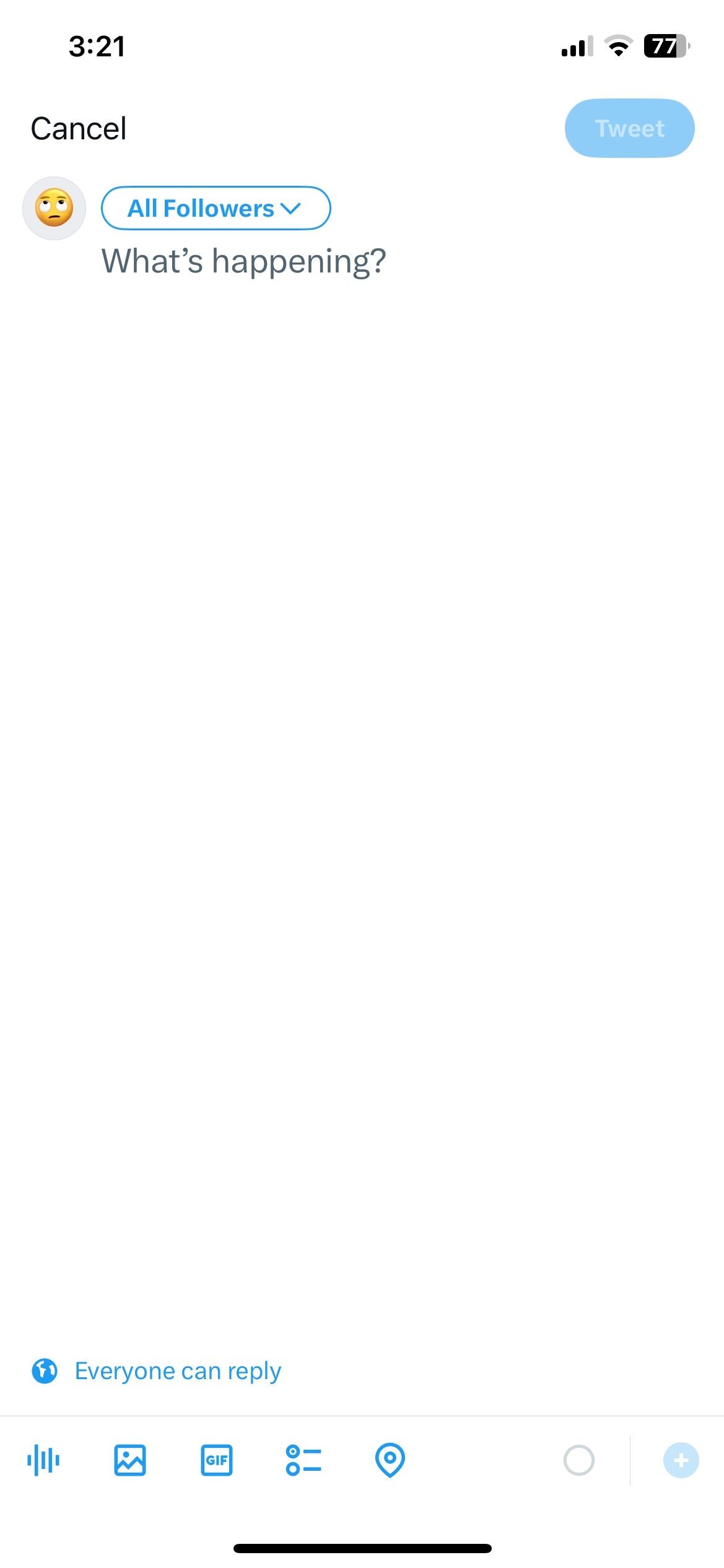A Twitter interface screenshot displayed on an iPhone shows a user composing a tweet. The tweet composition window is nearly empty, save for the text "What's happening?" addressed to all followers. A small, concerned emoji icon appears next to the text input area. The dropdown menu indicates that the tweet is intended for "Everyone," allowing all followers to reply. At the bottom, several interactive buttons are visible, including options to add a GIF, select a location, and access more tweet formatting features. The "Tweet" button in the top right corner is greyed out, indicating it is currently unclickable, and a "Cancel" button is located at the top left. The interface reflects the initial stage of engaging in a conversation on Twitter.